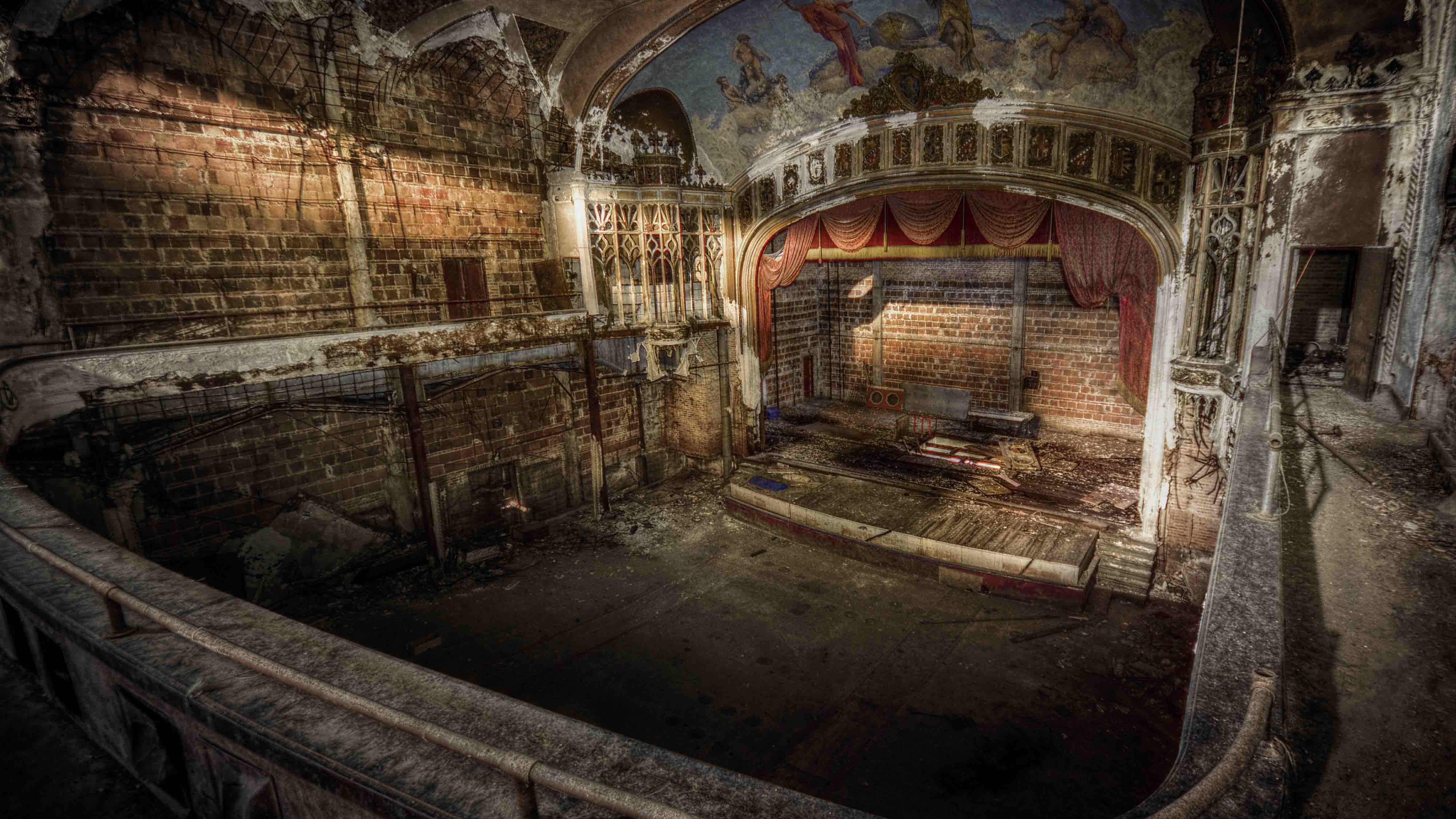This detailed photograph captures the haunting beauty of an abandoned theater, taken from the upper levels. The once-grand stage below now lies in ruin, featuring ragged red curtains still clinging to the archway, their vibrant color dulled and soiled by white mold. Once supported by interlocking wooden planks, the stage is now mostly pulled up, exposing large gaps and a sense of disrepair. The balcony offers a broader view, with a low railing topped with a dusty metal bar also covered in mold.

The bare brick walls of the theater are stark and imposing, their exposed surfaces marred by large patches of white mold. Ornate structures and decorative elements that might have adorned these walls have long since either rotted away or been stripped, leaving behind a sense of desolate beauty. Above the stage, a mural depicting various angels and robed figures amidst clouds adds a touch of faded glory. However, much of this elaborate painting has chipped away and succumbed to mold and decay.

The floor below, which once seated a lively audience, is now a barren concrete expanse littered with debris. A gray walkway, forming a U-shape around the stage, guides the eye through this scene of neglect. Despite the dire condition, or perhaps because of it, the abandoned theater radiates a melancholic charm, a testament to both its forgotten past and the relentless march of time.